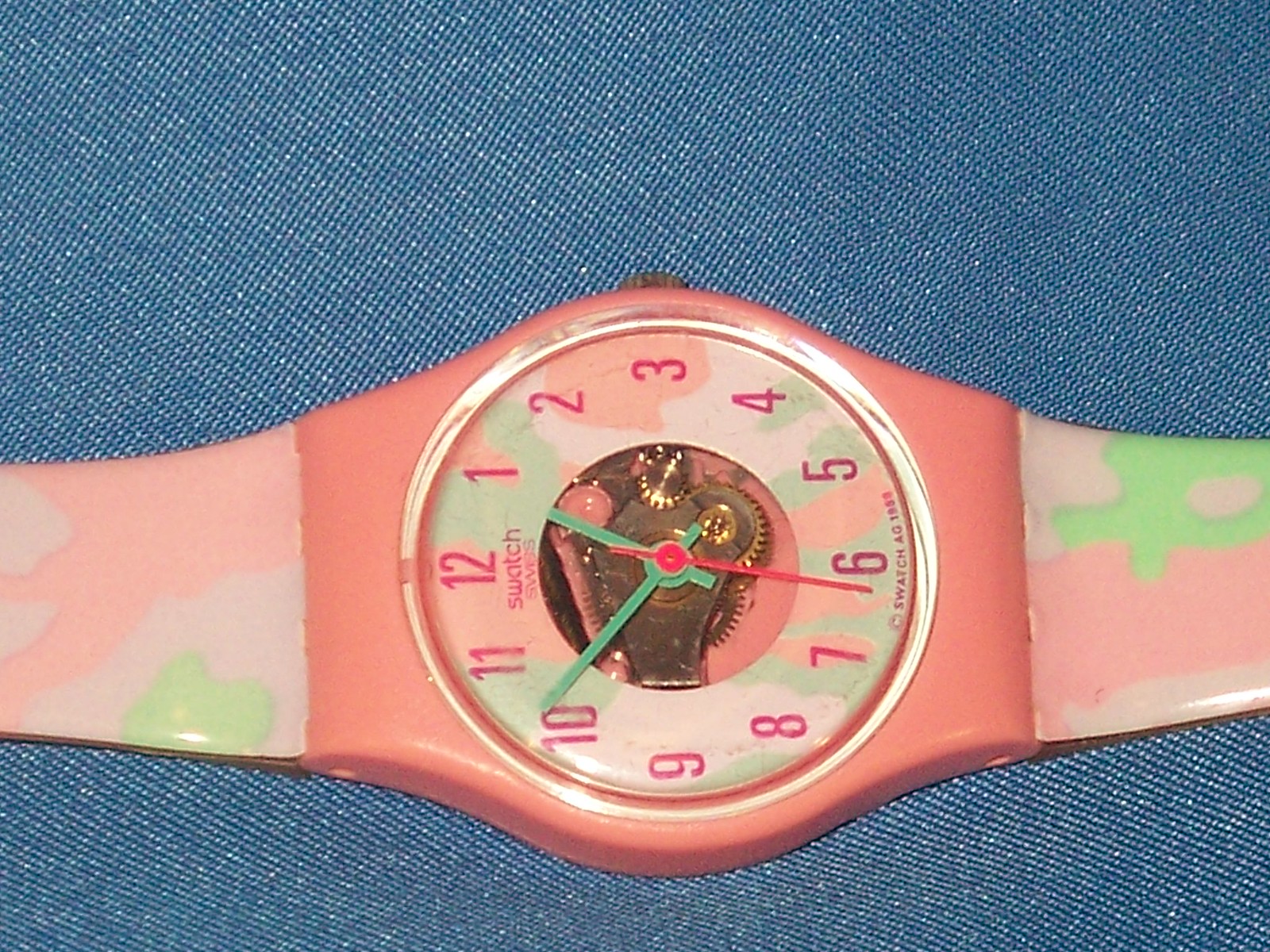This detailed image showcases a Swatch watch laying horizontally on a blue denim-like fabric, which closely resembles jean material. The watch is positioned with its 12 o'clock marker to the left and 6 o'clock to the right, requiring the viewer to turn their head sideways to properly orient the numbers. The vibrant watch features a plastic dark pink body and a colorful band with light pink, dark pink, green, and white shapes arranged in a camouflage pattern. The watch face is open in the center, revealing brass working gears inside. The time displayed is approximately eight minutes before 1 o'clock, indicated by green hour and minute hands and a red second hand marking around 32 seconds. The watch, identified as a Swatch, also has a button to set the time located towards the top.